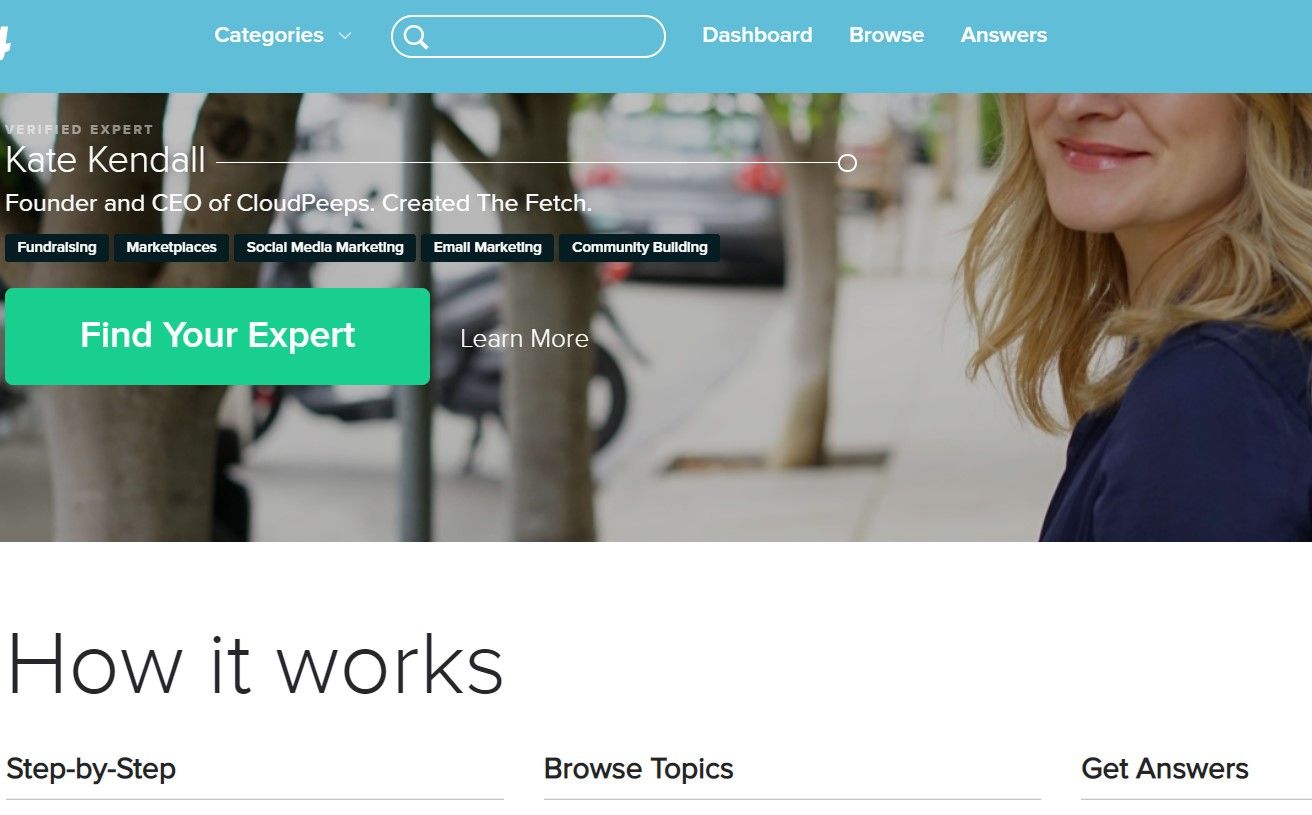This image depicts a webpage, likely a homepage or advertisement, arranged in a landscape orientation, making the photo much wider than it is tall. The page is rectangular and prominently features a white area alongside an image positioned in the upper half.

At the top of the webpage, there's a long rectangular bar with a light blue border. On this blue border, starting at the left edge, there's partially visible white text, followed by a white drop-down box labeled "Categories," a white search bar, and three navigation options titled "Dashboard," "Browse," and "Answers."

The background image displays a woman with blonde hair, smiling, and wearing a blue shirt, positioned towards the right-hand corner. She stands on a sidewalk, with cars and motorcycles parked behind her and trees lining the street in the background.

To the left of the image, small gray text reads "Verified Expert," followed by the name "Kate Kendall" written in large white letters. It notes that she is the Founder and CEO of CloudPeeps and that she created the fetch. Below her name, there are several black rectangular buttons with white text listing options such as "Fundraising," "Marketplaces," "Social Media Marketing," "Email Marketing," and "Community Building."

A green rectangular box with white text inside reads "Find your expert," followed by the call-to-action "Learn more." Below this section, in larger black letters, it states "How it works." There are headers indicating steps such as "Step-by-Step," "Browse Topics," and "Get Answers," suggesting a categorized guide or tutorial.